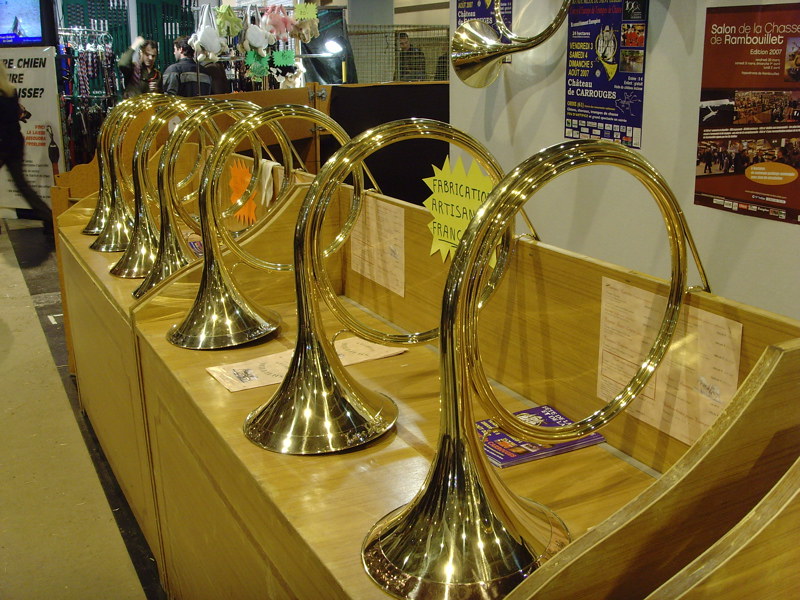This photograph captures a display of curved, horn-like musical instruments that resemble French horns or tubas, though they lack visible keys or buttons. The instruments are made of shiny, light metal and feature a large bell that curves into a big circular loop. Seven of these horns are lined up in a row, resting bell-down on a brown wooden display table that stretches diagonally from the upper left to the lower right of the image. The display table also features cabinets underneath and a partially visible yellow cardboard sign reading, "Fabrication Artisan France," along with some pamphlets scattered among the instruments.

Behind the table is a white wall adorned with posters, possibly related to music or concerts, and another horn is mounted on this wall. Towards the far left background, two men are engaged in conversation, with one of them raising his arm. Various items, such as stuffed animals and hanging bags, can be seen around the space, suggesting that the setting is a store selling a variety of goods. Additional details, like other items for sale and a couple of windows, are visible in the background, enhancing the sense of a bustling retail environment.